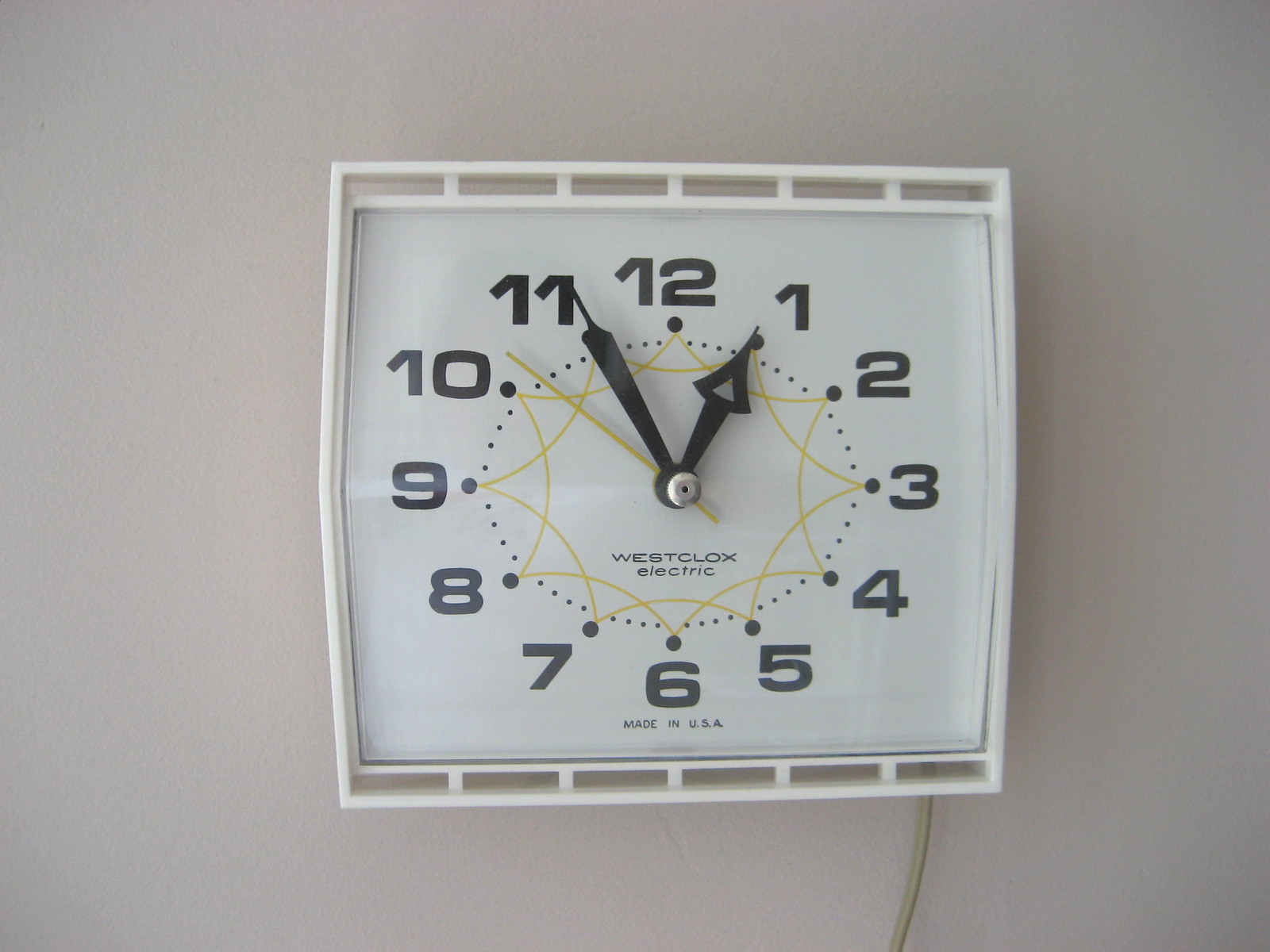This photograph captures a vintage, mid-century modern electric clock mounted on a pristine white wall. The square clock, featuring a round face encased in white plastic, exudes a timeless 1950s appeal. A cord trailing from the bottom right confirms its electric nature. Bold black numbers ranging from 1 to 12 encircle the dial, while the hour and minute hands, joined by a silver brad at their center, taper to pointed tips, resembling an arrow. Just above the number six, the brand "Westclox Electric" is prominently displayed. The clock’s face is adorned with a concentric circular pattern and a stylish yellow spirograph-like design at its center, adding an intricate touch to its classic look.